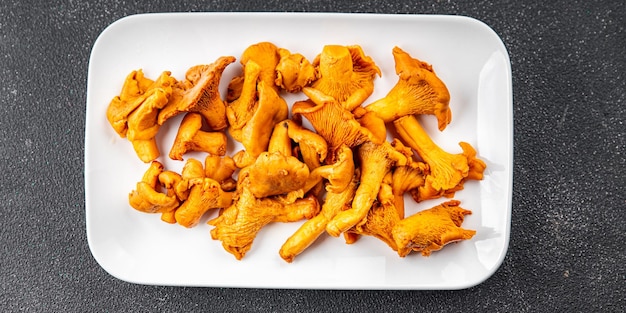The image depicts a long, rectangular, white plate with slightly rounded corners and a shiny surface, sitting on a gray countertop speckled with white, possibly granite or asphalt. The plate is not completely flat but has a slight concavity, especially visible on the right side where light creates a subtle shine. It is piled with numerous mushrooms, both caps and stems, which range in color from brown to orange and appear fried or dried. The background of the image shows a rough and varied texture, with more pronounced white specks and scuff marks on the right side of the countertop, giving way to smoother areas with smaller white specks and possible water spots on the left side.